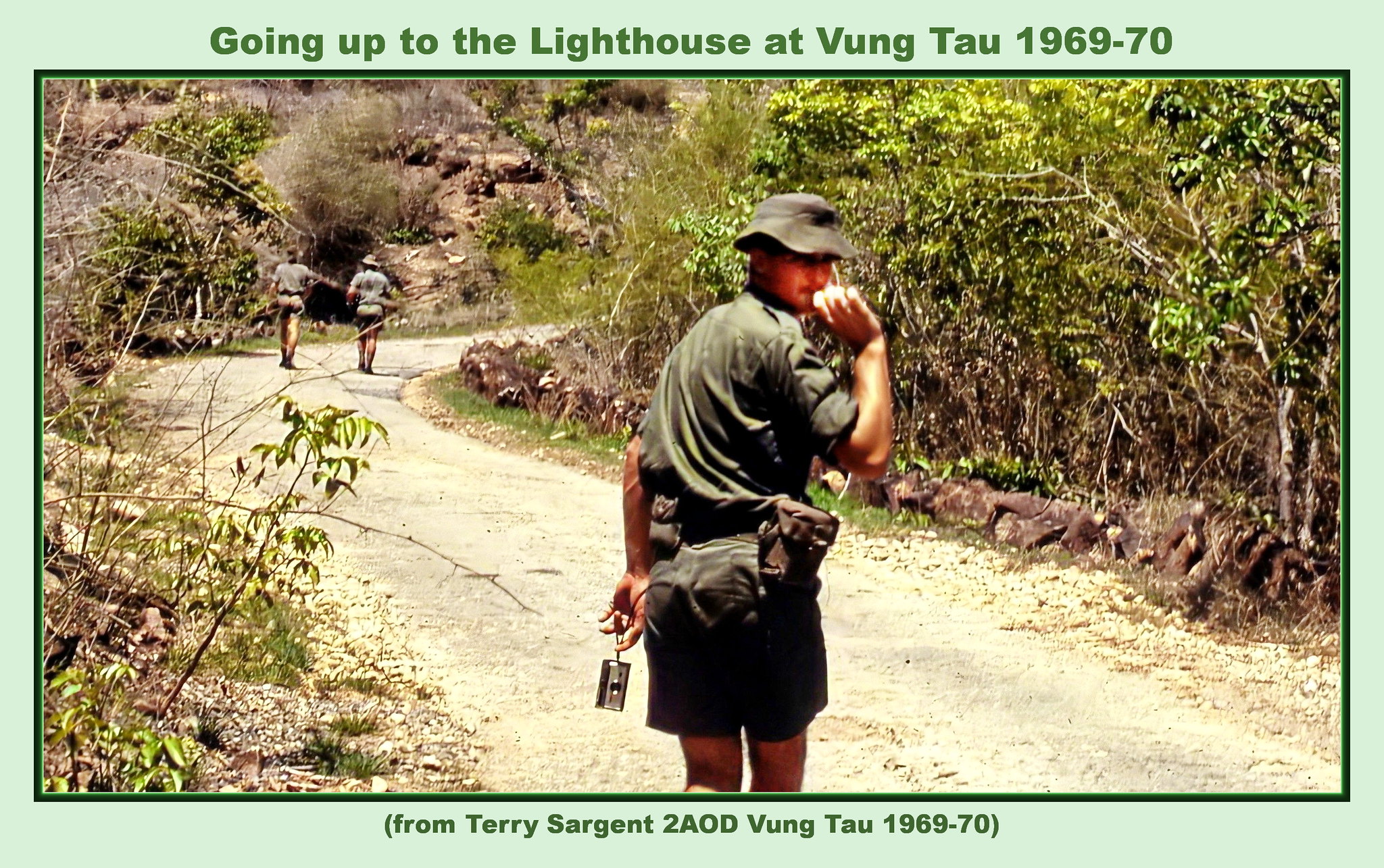This vintage-style color photograph, inset into a light green background, features a man on a dirt path flanked by woods on both sides. He is wearing a green military-style cap, a green shirt, olive pants, and two belt bags on his waist. Positioned facing away from the viewer, he glances over his right shoulder with his hand to his chin, while a camera dangles from his left wrist. In the distance, two similarly dressed individuals can be seen walking further along the path, which curves and disappears around a bend with mountains visible in the background. The photograph is bordered by a dark green rule, with a headline at the top reading "Going up the lighthouse at Vung Tau 1969-70" and a caption at the bottom, in dark green text, stating "(from Terry Sargent to AOD Vung Tau 1969-70)." The overall style evokes a vintage photography graphic design.